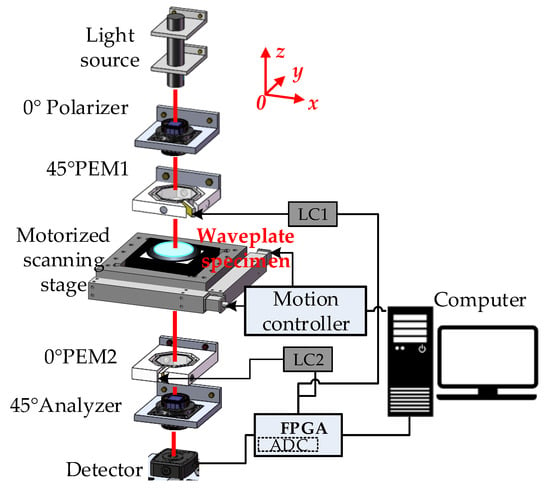The image appears to be a detailed illustration, possibly from a textbook or instruction manual, showcasing the internal components and connections of a computer system or technological device. The illustration features a white background with no borders, and it prominently displays various silver pieces interconnected by red lines. On the right side of the image, there is a depiction of a computer, including a screen and a tower. 

Text along the left-hand side of the illustration lists the components in a top-to-bottom sequence: "Light source, zero-degree polarizer, 45-degree PEM1, motorized scanning stage, zero-degree PEM2, 45-degree analyzer, and detector." There are accompanying images illustrating these components. 

A prominently labeled red arrow, originating from a point marked zero and branching off toward Z, Y, and X axes, indicates the coordinate directions. Another red label reads "wave plate specimen." In a separate section, additional components are noted: "LC1, motion controller, LC2, and FPGA ADC," with red lines connecting all elements. The word "computer" helps to orient the viewer, suggesting these components integrate or interface with the computer. The overall diagram provides a systematic visualization of how these elements are interconnected, effectively guiding the reader through the inner workings of the system.